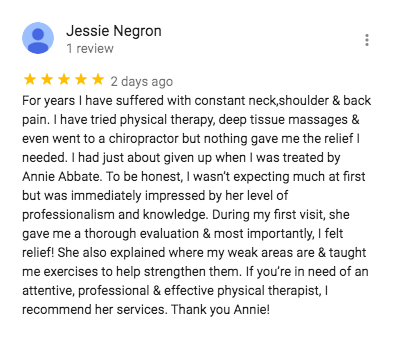The image is a screenshot of an Amazon.com review for a product, framed in a square format where the top, bottom, left, and right borders are of equal length. The review is presented against a white background with multiple lines of black text. At the very top, the text reads "Jesse Negron," indicating the reviewer's name, accompanied by a blue avatar or circle with a user illustration to the left. Below the name, it shows that this is Jesse's one review, followed by five yellow stars, indicating a five-star rating, and the words "two days ago" next to the stars.

The main body of the review details Jesse's experience, starting with, "For years I have suffered with constant neck, shoulder, and back pain. I have tried physical therapy, deep tissue massages, and even went to a chiropractor, but nothing gave me the relief I needed. I had just about given up when I was treated by Annie Abate. To be honest, I wasn't expecting much at first but was immediately impressed by her level of professionalism and knowledge. During my first visit, she gave me a thorough evaluation and most importantly, I felt some relief. She also explained where my weak areas are and taught me exercises to help strengthen them. If you're in need of an attentive, professional, and effective physical therapist, I recommend her services. Thank you, Annie."

The overall impression given is that of a highly positive, detailed, and personal review emphasizing the effective treatment and professional service provided by Annie Abate.